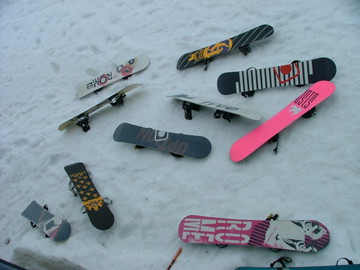The photo showcases an array of roughly ten snowboards scattered on a blanket of powdery white snow, which is peppered with footprints weaving in and around the boards. The snowboards, predominantly black with different decals, display a vivid assortment of colors and patterns. Among them, one snowboard is strikingly pink, another features white and black horizontal stripes, while yet another is adorned with yellow polka dots on a black background. Additionally, there are gray boards with diagonal tiles and a couple of white ones. The boards vary in size, with a particularly short one at the bottom left and several longer ones positioned at the top and bottom right. Each snowboard lies upside down, revealing their bindings and decals, with no wheels to be seen, contradicting any mention of skateboards. In the bottom part of the photo, the edge of a ski lift looms, adding context to this vibrant assembly of snowboards.